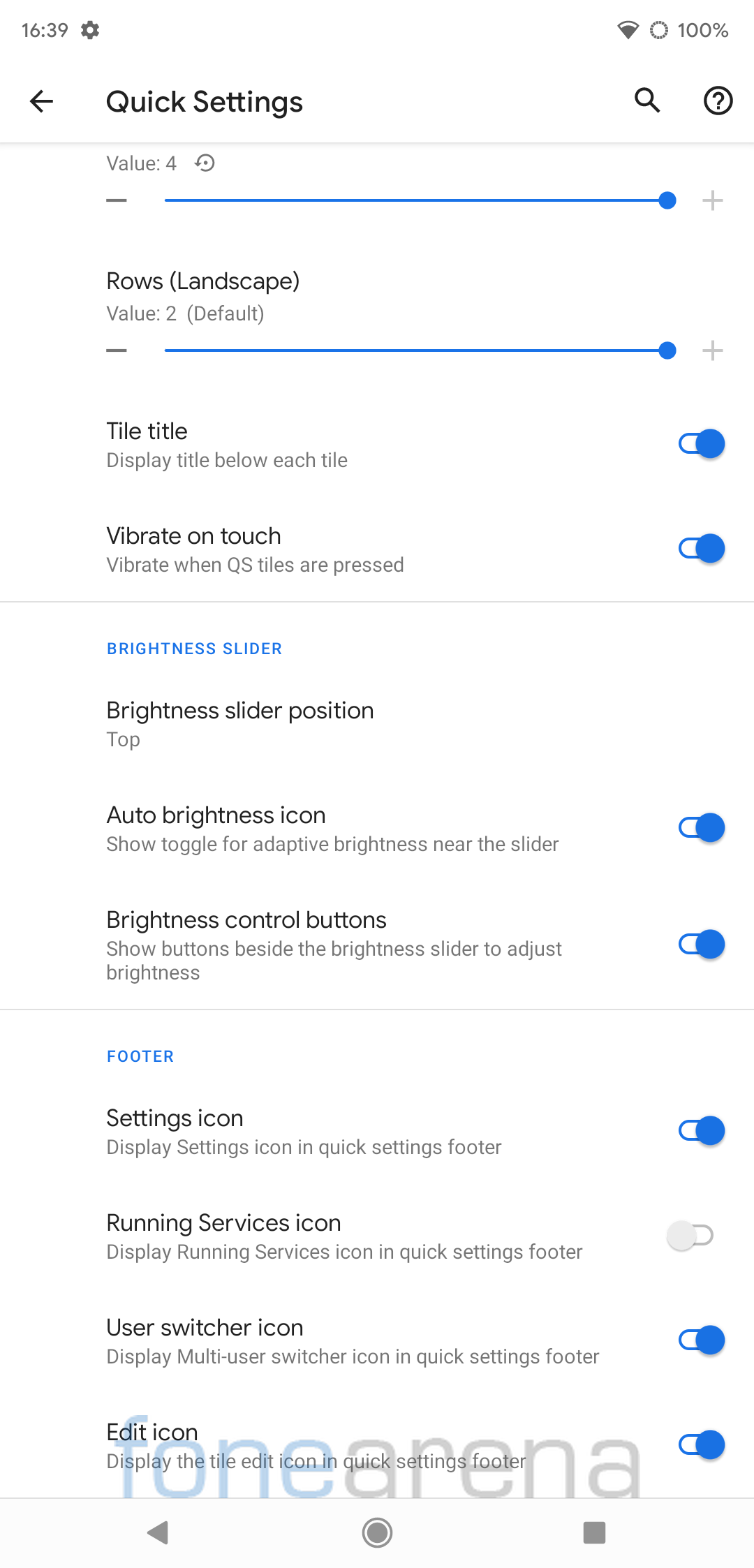The upper left corner of the image displays the time "16:39" next to a gear shift icon. On the right side, there is a downward-pointing triangle, rounded at the top, partially filled in with gray. Below this, a gray-outlined circle contains the text "100%". Additionally, an arrow points leftwards to text that reads "Quick settings". On the far right, there is a magnifying glass icon and a circle with a question mark inside it. 

A pale gray line runs beneath this section, followed by text that says "Value: 4" next to a circular arrow icon. Below, a short gray line precedes a long blue line capped with a blue dot. To the right of this, a light gray plus sign appears next to the text "Rose (Landscaping Value: 2) (Default)". 

Another short gray line extends below this, leading to another long blue line ending in a blue dot, with a gray plus sign next to it. The text "Title" is displayed, with "Tile title" and "Display title below each line" located alongside it. On the right, a blue lock icon accompanies the text "Vibrate to touch" followed by more descriptive text.

Further down, the image shows additional blue lock icons beside settings related to brightness. Phrases include "Brightness sliders", "Brightness slider position at top", "Auto brightness", and "Brightness icon". Below this section, more text describes brightness-related settings, again accompanied by blue lock icons.

Another gray line appears, marked with the text "Footer setting icons" followed by more text and a blue lock icon. Below this, "Running service icons" and another gray lock (pointing in the opposite direction) are displayed alongside "Use switcher icon" and more descriptive text.

At the bottom, blue lock icons accompany phrases such as "Edit icon" and other indistinguishable text. In the background, a final segment includes the text "Phone Arena", an arrow pointing left, a gray-outlined circle with a central gray circle, and a gray rectangle or square.